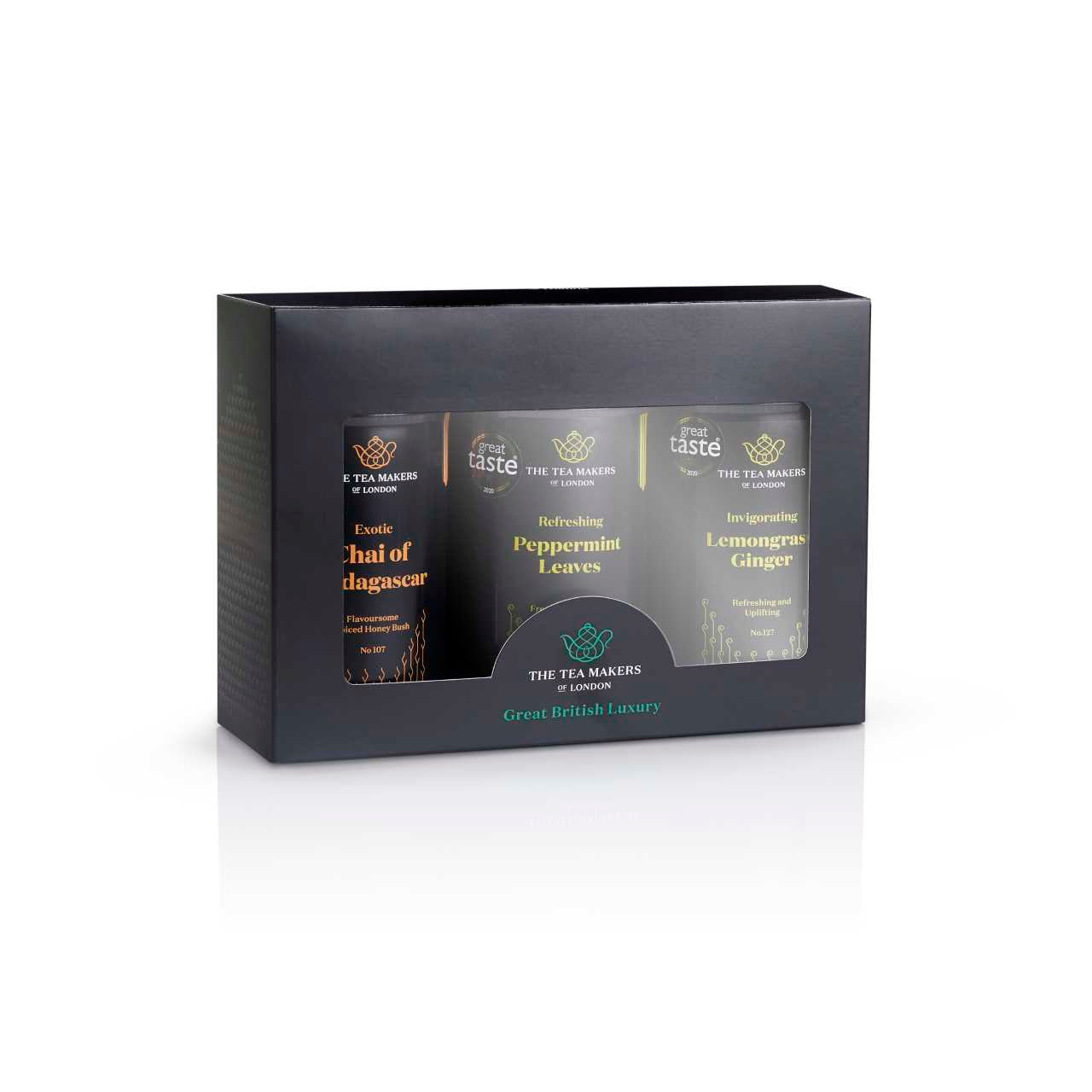This detailed photograph showcases a luxurious tea set from the renowned Tea Makers of London, emphasizing the sophisticated nature of British luxury tea. The set consists of three distinctive tea varieties housed in elegant matte black containers, all neatly arranged in a stylish black box. The box features a transparent plastic window in the center, allowing a clear view of the teas. From left to right, the varieties included are:

1. **Exotic Chai of Madagascar**: Presented in a black and orange container, this chai boasts flavorsome spiced honeybush, infusing a rich, aromatic experience.
  
2. **Refreshing Peppermint Leaves**: Housed in a black container with green accents, it offers a cool and invigorating flavor, though the full text is obscured by the front logo.

3. **Invigorating Lemongrass Ginger**: Packaged in a black and yellow container, it promises a refreshing and uplifting experience.

The packaging is meticulously designed, with the brand name, "The Tea Makers of London," displayed in white text at the bottom, and an elegant tagline, "Great British Luxury," written in green. The clear cover elegantly reveals the trio of tea containers, each distinctly labeled and colored to denote their unique flavors.